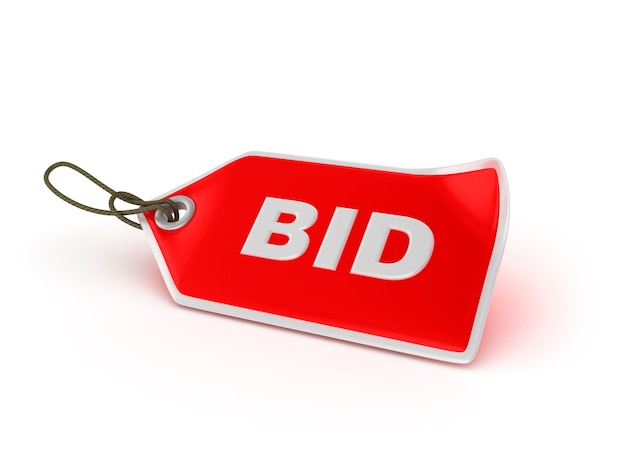In the image, there's a striking red tag prominently positioned against a pure white background. The tag itself has a unique shape: it's mainly rectangular, but the left side tapers into a triangular point. This pointed end features a metallic ring with a piece of string threaded through it, allowing the tag to hang. The tag is adorned with a thin white border that outlines its entire perimeter. In the center, large white capital letters spell out the word "BID." Additionally, the tag's upper right corner appears to be bent upwards, adding a subtle detail to its design. A light red drop shadow behind the tag provides a sense of depth against the white backdrop.